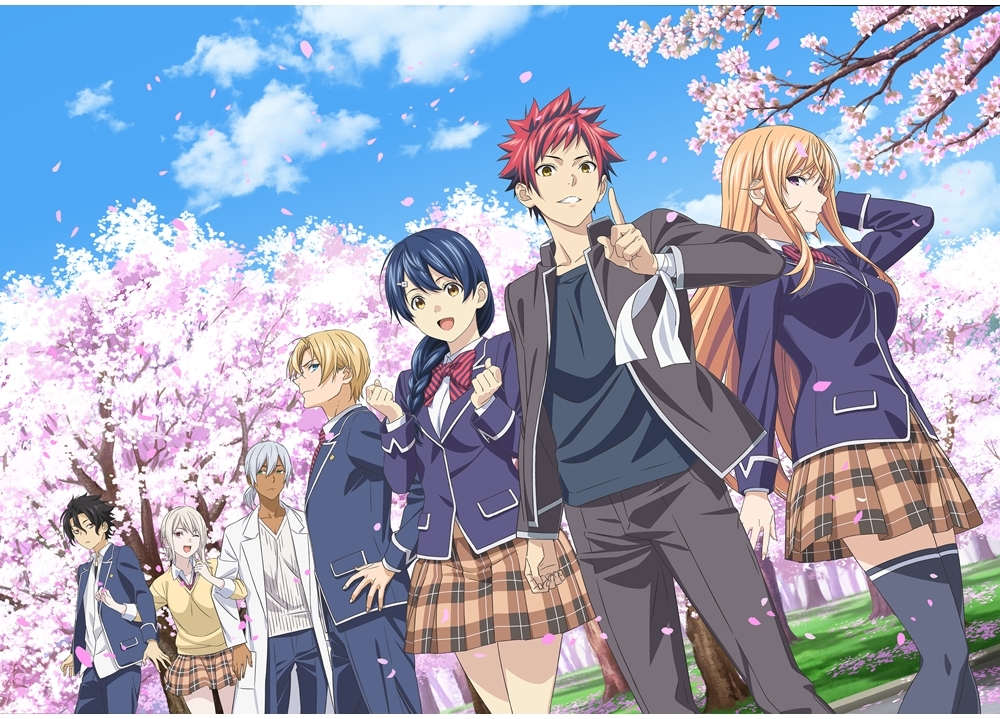This image features seven anime characters positioned in a staggered formation, taken at an angle that creates a layered effect. The four characters in the front are closest to the camera, with the remaining three slightly obscured behind them.

Starting from the right, the first character is a female with her head turned, providing a view predominantly of her right profile. She is dressed in a brown plaid skirt and a blue top. Next to her stands a male character with spiky red hair. To his left is another female character, who faces the camera directly. She is also wearing a brown plaid skirt and a blue top, complemented by a red, scarf-like bow tie. Her mouth and eyes are wide open, suggesting a state of surprise or excitement. Completing the row of four in the front is a male character on her left, who is turning toward the left side. The intricate detail in their attire and expressive facial features make the characters vibrant and engaging.